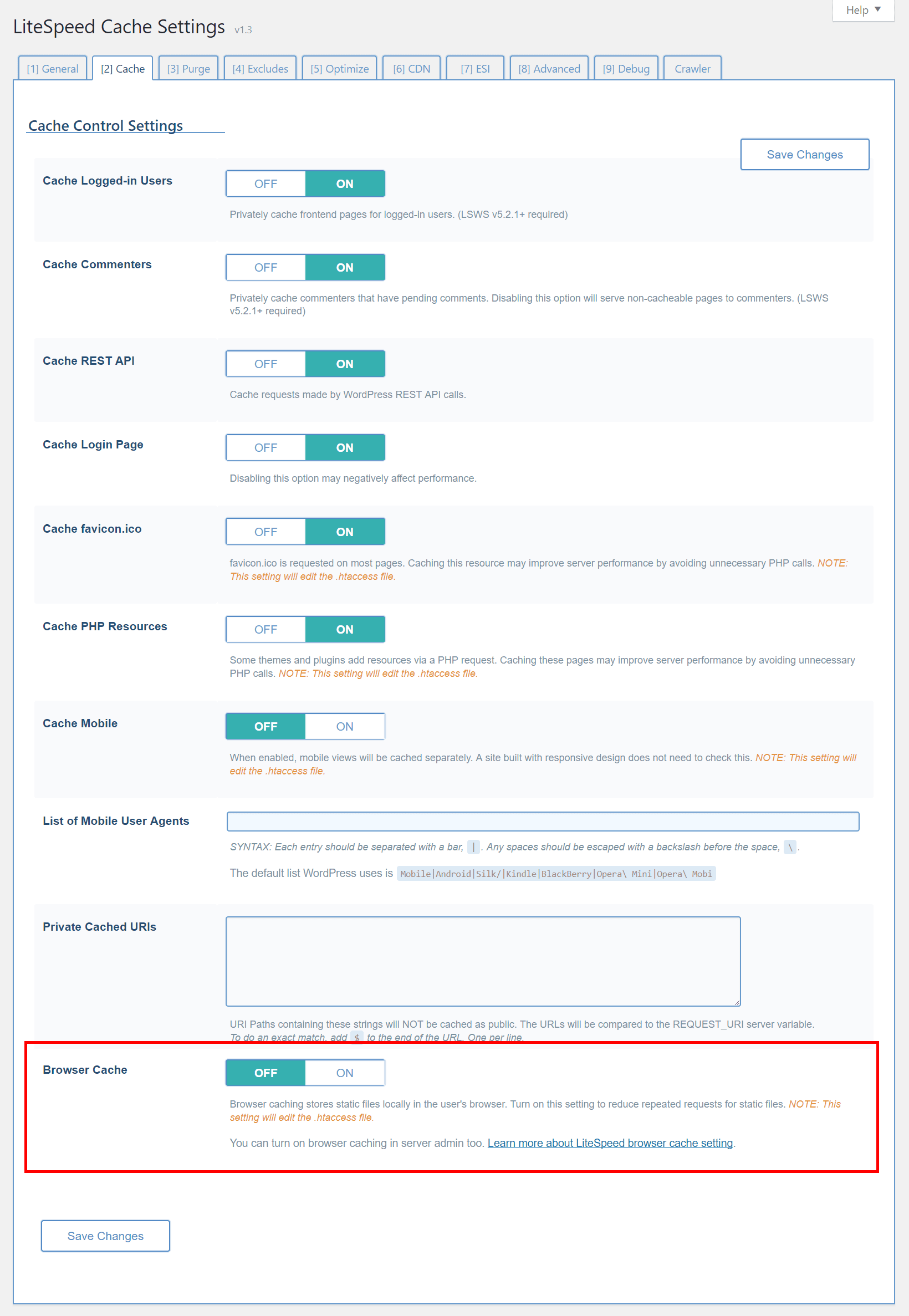This image depicts the Light Speed Cachet Settings tab within a software interface. At the top-left corner, the header reads "Light Speed Cachet Settings" in small black letters. On the far right of the same horizontal bar, there's a small drop-down box with a white background. 

Beneath this, a row of ten horizontally-aligned tabs is visible, each thinly outlined in blue. The second tab, labeled "Cachet," is selected, displaying its corresponding options on a white background.

Below the tabs, on the top left, the text "Cachet Control Settings" appears in blue. Following this, a vertical list of on/off toggle options is visible. Every option except the last one, "Cachet Mobile," is toggled on. 

At the very bottom of the screen, the text "Discover Cachet" is displayed in red, with a red box around it, and this option is toggled off. To the bottom right, a prominent white button labeled "Save Changes" invites the user to save their adjustments.